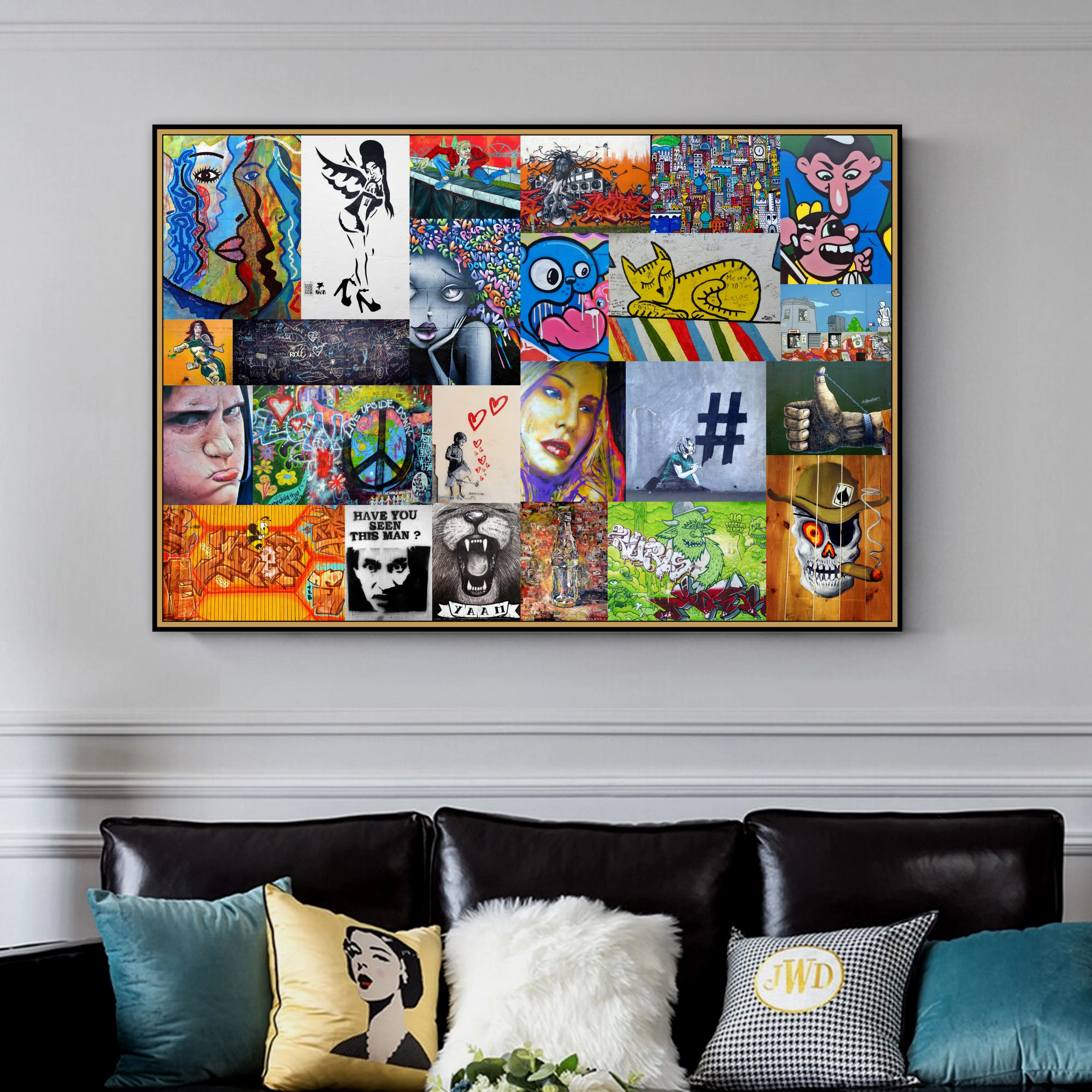This image depicts a cozy living room with a clearly modern, eclectic style. Central to the composition is a black leather couch with squared armrests, sporting a variety of five decorative pillows. At either end of the couch are teal pillows, bringing a pop of color to the room. In the middle, there's a white furry pillow flanked by a yellow pillow featuring a retro pop art image of a woman's face with red lipstick reminiscent of 1950s magazine covers, and a houndstooth pillow with the initials "JWD" in a white oval, with the 'W' notably larger. The couch is placed against a white wall with a chair rail trimming. Adorning the wall above the sofa is a large, framed print resembling a vibrant mosaic of overlapping postcards. This intriguing artwork includes colorful elements such as cartoon characters, human portraits, and a skull with a cigar, all arranged in a meticulous yet lively fashion. The poster's palette features blue, yellow, red, orange, and black hues, further enhancing the room's dynamic atmosphere.